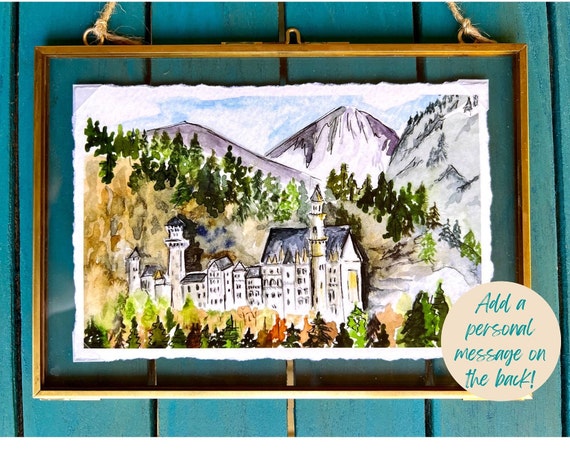This advertisement features an artistic painting presented in a gold-framed picture hanger, set against a turquoise blue wooden wall that resembles a picket fence with visible gaps in between the slats. The frame, designed with two pieces of clear glass, allows you to see through to the rough-edged watercolor painting inside, which depicts snow-capped mountains, verdant green trees, and a valley with several buildings, including a prominent three-story cathedral-like structure. The frame is secured with two eye hooks and twine, and it boasts silver corner covers and a small gold hinge at the center for easy picture replacement. In the bottom right corner, a white circle with blue cursive text reads "add a personal message on the back," emphasizing customization. The detailed landscape scene, complete with blue skies and hints of orange foliage, is a beautiful, customizable piece of art available for purchase.